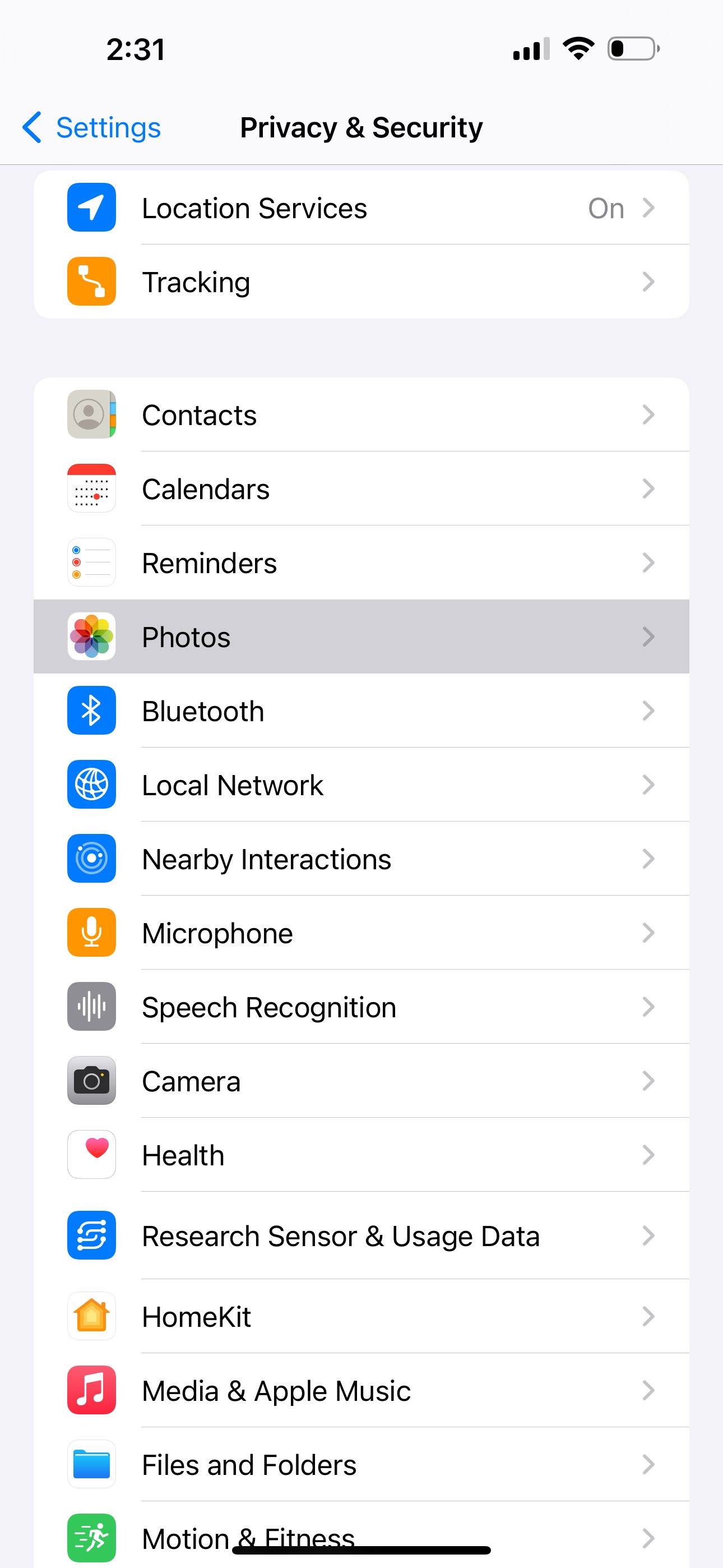The image showcases a screenshot of a smartphone displaying the "Privacy and Security" settings section. The phone's status bar is visible at the top of the screen. On the top right, there's a battery icon indicating the phone's charge level next to a mostly white background, with a small amount of black on the far left. To the left of the battery icon is a full Wi-Fi signal symbol. Continuing left, there's a phone signal strength indicator showing 3 out of 4 bars filled in black. At the top left corner, the time is displayed as 2:31.

Beneath the status bar, centrally aligned, the heading "Privacy and Security" is visible. Left of this heading, the word "Settings" appears. As the image progresses downward, a series of privacy and security settings are listed vertically:

1. Location Services - indicated as 'On'
2. Tracking
3. Contacts
4. Calendar
5. Reminders
6. Photos
7. Bluetooth
8. Local Network
9. Nearby Interactions
10. Microphone
11. Speech Recognition
12. Camera
13. Health
14. Research Sensor
15. HomeKit
16. Media
17. Files and Folders
18. Motion and Fitness